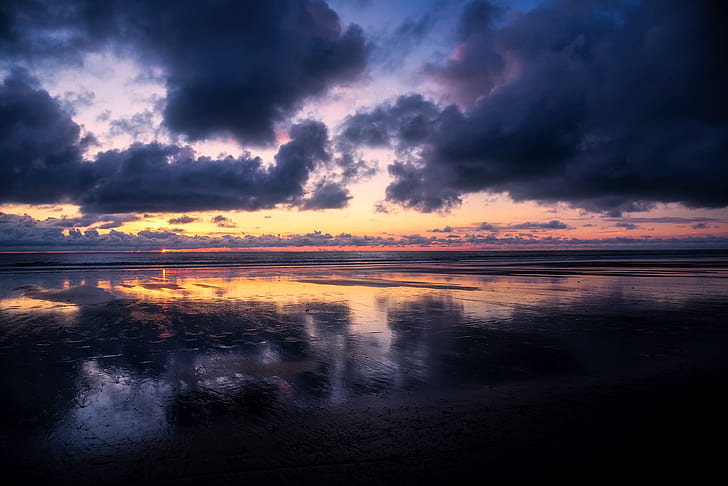This photograph captures a moody, atmospheric sunset over a beach, with dark, stormy clouds dominating the upper portion of the scene and just a hint of clear sky peeking through. The sunset, though barely visible as a small glint on the middle left, paints the entire landscape in deep, saturated hues of oranges, yellows, and pinks, contrasting against the dark blues and grays of the clouds. The sand and wet shoreline mirror the dramatic sky, appearing almost black with glistening reflections of the sky's colors. The image's expanse, spanning the whole page, draws the eye from the tumultuous clouds above to the reflective, shadowed beach below, creating a sense of depth and endless horizon.